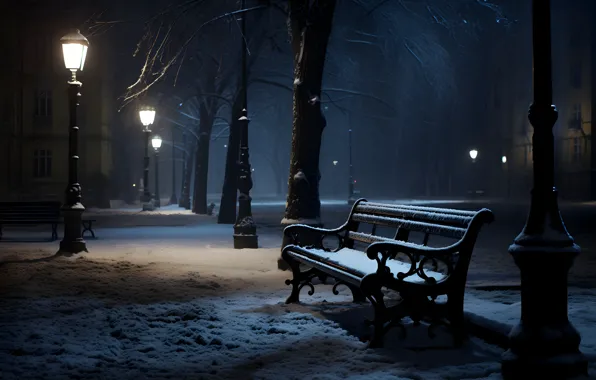The nighttime scene captures a serene city street blanketed in snow. The street is lined with old-fashioned, black wrought iron street lamps that emit a soft glow, casting delicate light onto the snow-covered sidewalk and the bare tree branches, which arch gracefully over the street. In the foreground stands a park bench, distinct with its wrought iron ends and timber slats, also covered in snow, positioned between a lamppost and a medium-sized tree. The opposite side of the street mirrors this setup with similar lamps and trees, while across the street are snow-laden, leafless trees and what appear to be apartment buildings. The quietness of the empty, wide street with no cars or people in sight accentuates the peaceful, almost nostalgic ambience of this wintery urban nightscape.